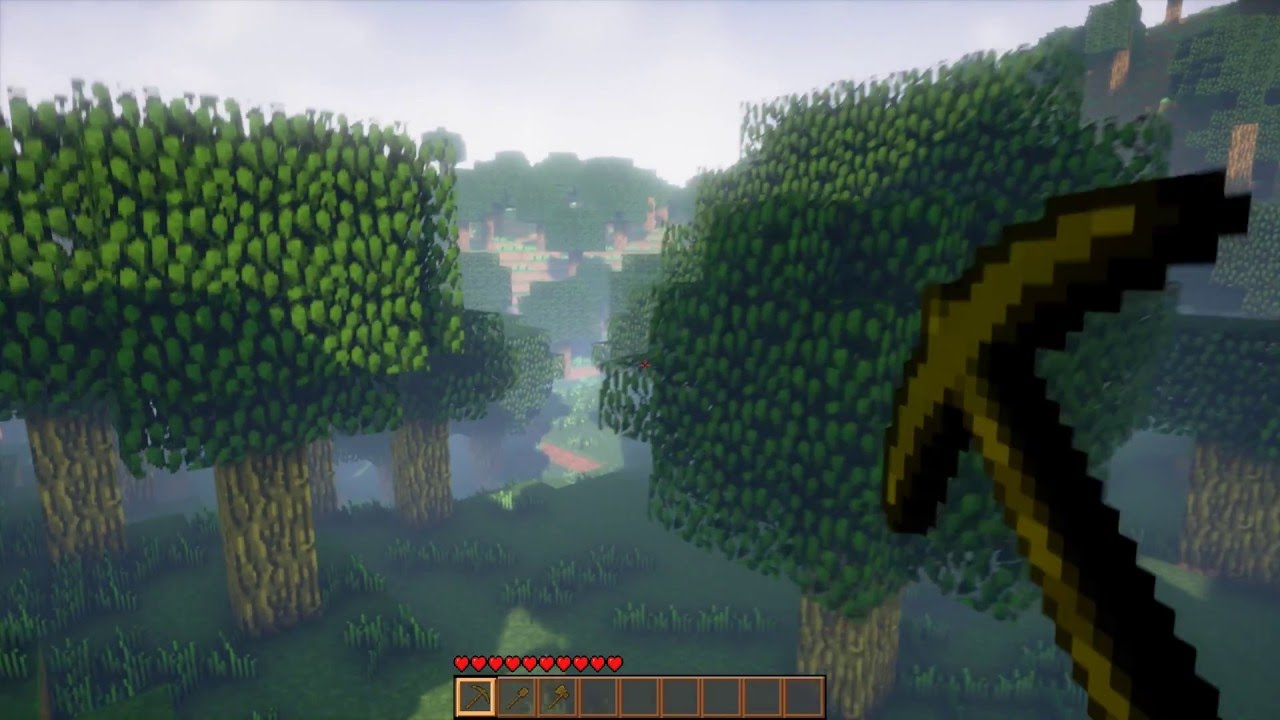This detailed screenshot of a video game closely mimics the visual style of Minecraft. The image is rendered in a first-person perspective, where the player character wields what appears to be a pixelated axe. Despite the simplistic, bitmap-like graphics, the game maintains a modern quality.

At the bottom of the screen, there's a status bar indicating the player’s currently selected item, with the pickaxe highlighted among three available tools. A health bar featuring ten fully red hearts is also visible, signifying full health.

The landscape includes well-defined, blocky trees and pixelated grass, with surrounding mountains covered in green foliage. The backdrop displays a clear blue sky, which contributes to the blend of nostalgia and contemporary design elements.